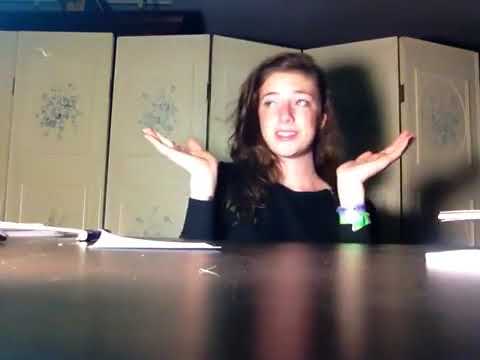In this indoor setting, the subject is a teenage girl, around 13 years old, seated at a dark brown wooden table covered with paperwork, including a piece of paper to her right and a stack of softcover books or binders to her left. The girl, with long dark brown hair parted on the side, is wearing a black long-sleeve shirt and a bracelet on one wrist. She sits with her hands raised to chin level, palms facing upwards, as if expressing surprise or exasperation, and gazes slightly to the left, not directly into the camera. Behind her is an older, somewhat worn multi-panel accordion-type screen with a beige fabric featuring blue floral motifs. The photograph is in landscape orientation and is a realistic, representational depiction of the scene.